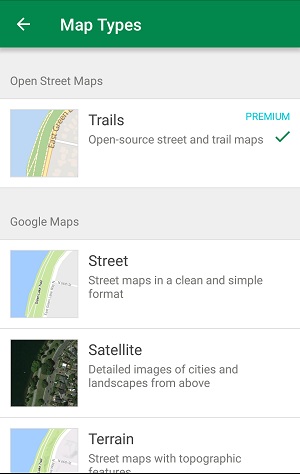This screenshot showcases a selection interface for different map types. At the top, a green banner prominently displays the title "Map Types." Directly beneath it, a light blue banner labeled "Open Street Maps" is featured. Below this banner, there is a small map labeled "Trails," accompanied by the text "Open Source Street and Trail Maps." To the right of this description, the word "Premium" is displayed in blue letters, alongside a checkmark indicating that it is a selected option.

Further down, another blue banner introduces "Google Maps" with three distinct choices listed below:

1. **Street**: Street Maps in a clean and simple format.
2. **Satellite**: Detailed Images of Cities and Landscapes from Above.
3. **Terrain**: Street Maps with Topographic Features.

The interface allows users to choose between these various types of maps, with the "Premium" option providing access to higher quality, open-source street and trail maps. The Google Maps choices offer standard formats, including street-level views, satellite imagery, and topographic maps, catering to different user preferences and needs.